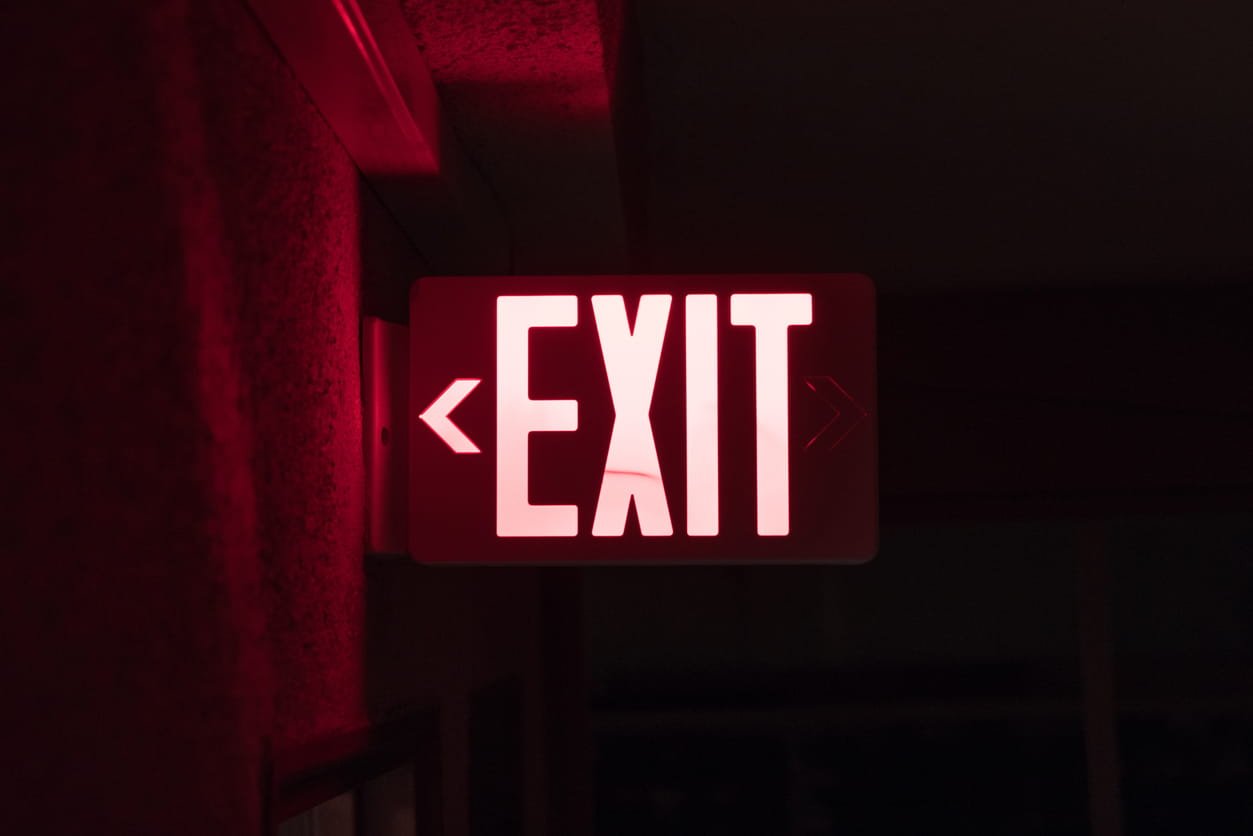The image is a simple, straightforward one-color photograph taken indoors using artificial lighting. It prominently features an EXIT sign, which is brightly lit in red and situated in the center of the photograph. An arrow on the sign points to the left. Surrounding the sign, the background is predominantly dark, almost black on the right side, while there is a reddish glow emanating from the sign itself on the left side. The sign’s illumination gently lights up the wall behind it, creating a noticeable contrast. Below the sign, there is a hint of a doorway frame, suggesting an exit path, but the rest of the scene fades into darkness, making other details nearly imperceptible. A faint outline of what could be a shelf appears in the bottom right, though it remains obscure. The photograph is horizontal and rectangular in shape, focusing solely on the EXIT sign against the dark background.